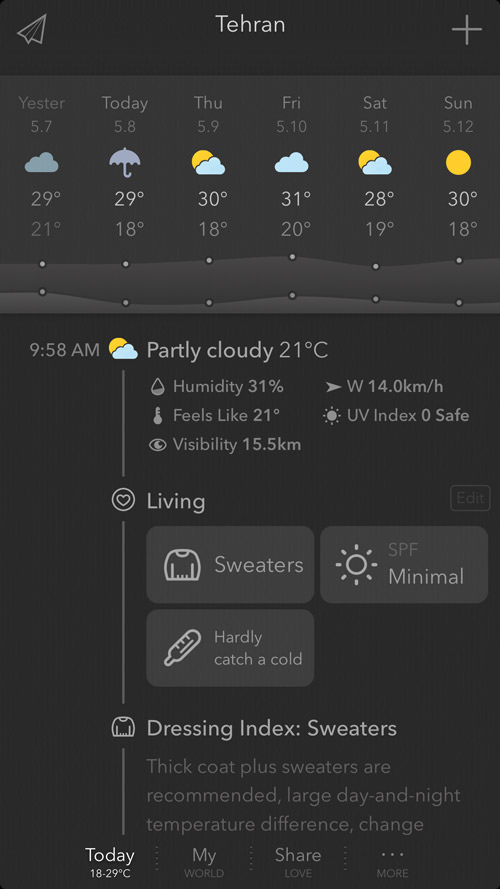Screenshot of Tehran Weather Forecast

This detailed screenshot from a weather application shows the forecast for Tehran with the current date and time being 9:58 AM. The city is Tehran, and the current weather is partly cloudy with a temperature of 21°C. The following information is provided for the forecast:

- **Current conditions:**
  - Temperature: 21°C (Feels like 21°C)
  - Humidity: 31%
  - Wind: West at 14 km/h
  - Visibility: 15.5 kilometers
  - UV index: 0 (Safe)
  - Suggested clothing: Sweaters
  - SPF: Minimal
  - Health indication: Hardly catch a cold; Thick clothes and sweaters are recommended due to a large day and night temperature difference.

- **Previous and upcoming forecasts:**
  - **Yesterday:** High of 29°C, Low of 21°C, Partly cloudy
  - **Today (5/8):** High of 29°C, Low of 18°C, Rainy
  - **Thursday (5/9):** High of 30°C, Low of 19°C, Partly cloudy
  - **Friday (5/10):** High of 31°C, Low of 20°C, Cloudy
  - **Saturday (5/11):** High of 28°C, Low of 19°C, Partly cloudy
  - **Sunday (5/12):** High of 30°C, Low of 18°C, Sunny

At the bottom of the screenshot, options for "Today" are highlighted with temperatures ranging from 18°C to 29°C. Additional features such as "My World," "Share," "Love," and "More" (three dots) are visible, maintaining a typical layout for weather and health-related indications.